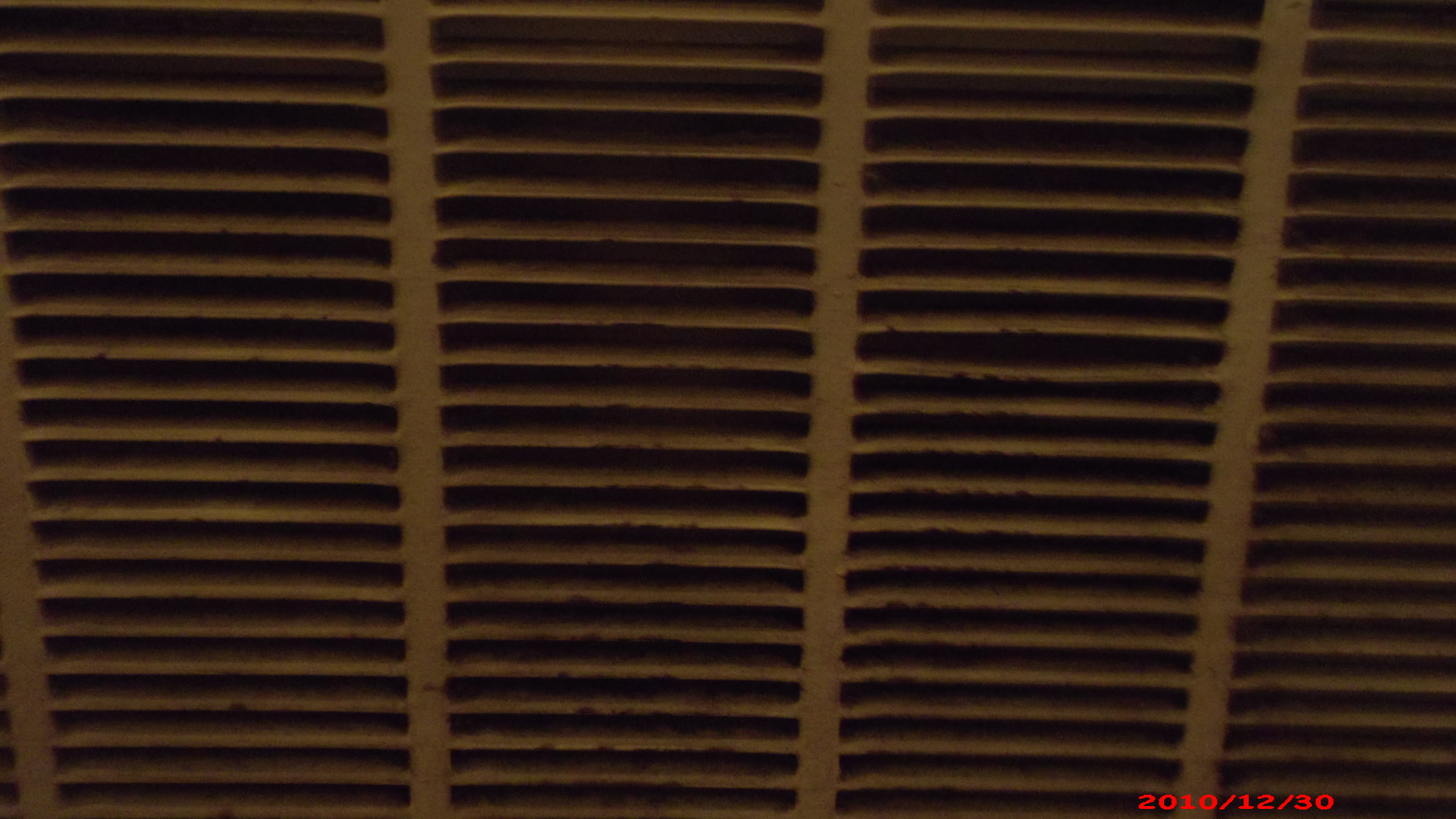The image depicts a somewhat old and rusting air vent, primarily metallic and white in color, with noticeable rust and dirt on the horizontal bars. The vent structure consists of four vertical bars and 20 horizontal bars. At the bottom right corner of the photograph, there is a timestamp reading "2010-12-30," indicating the date it was taken. The vent likely serves to release air, possibly from an air conditioning or heating system, or even from an oven or refrigerator.